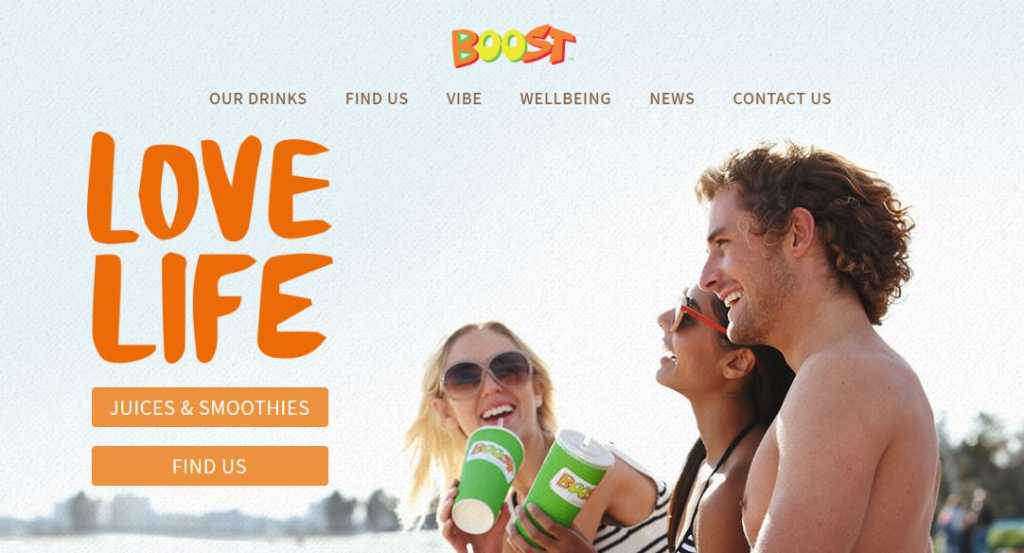The image is a horizontal screenshot of an advertisement for the brand Boost, characterized by a cartoon-style typeset in vibrant orange, green, and yellow colors, positioned prominently at the top center. The photograph, which occupies the entire background, depicts a summer beach scene with a very pale blue sky.

At the top of the image, there are six navigation buttons labeled "Our Drinks," "Find Us," "Vibe," "Wellbeing," "News," and "Contact Us," representing different sections of the website. On the left side of the screen, in large, orange bubble type, the text "Love Life" is displayed with "Love" above "Life." Below this slogan, two orange buttons provide further options, labeled "Juices and Smoothies" and "Find Us."

The image features three people enjoying a sunny day at the beach, all smiling and laughing. Two of the individuals are drinking Boost smoothies from green cups with white lids and straws. Among the group, there is a woman with blonde hair, a woman with brown hair wearing red sunglasses, and a man with brown hair. The scene exudes a joyful, carefree vibe, perfectly encapsulating the brand's lively and positive attitude.